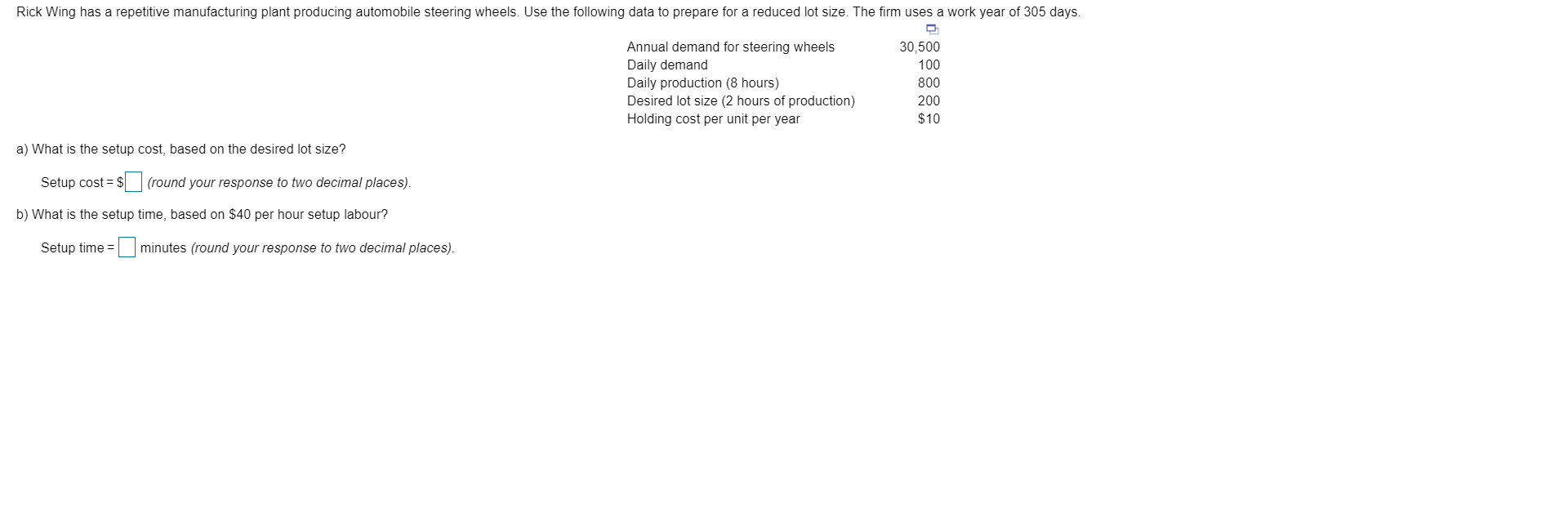This screenshot depicts a cost calculation interface for automobile steering wheels, displayed on a plain white background. At the top, it states, "Rick Wing has a repetitive manufacturing plant producing automobile steering wheels. Use the following data to prepare for reduced lot size. The firm uses a work year of 305 days." Directly beneath this text, on the right-hand side, there are small icons. Below the icons, are the following details: 

- Annual demand for steering wheels: 30,500 units
- Daily demand: 100 units
- Daily production: 8 hours, 800 units
- Desired lot size: 2 hours of production, 200 units
- Holding cost per unit per year: $10

To the left, two questions are presented:

**Question A:** "What is the setup cost based on desired lot size?" This is followed by the prompt "Setup cost equals" and an input box, with a note instructing users to "round your response to two decimal places."

**Question B:** "What is the setup time based on $40 per hour setup labor?" This is followed by the prompt "Setup time equals" and an input box, with a note indicating the input should be in minutes.

This detailed interface provides essential data and structured questions to determine the cost implications and time requirements for setting up production batches in the manufacturing plant.